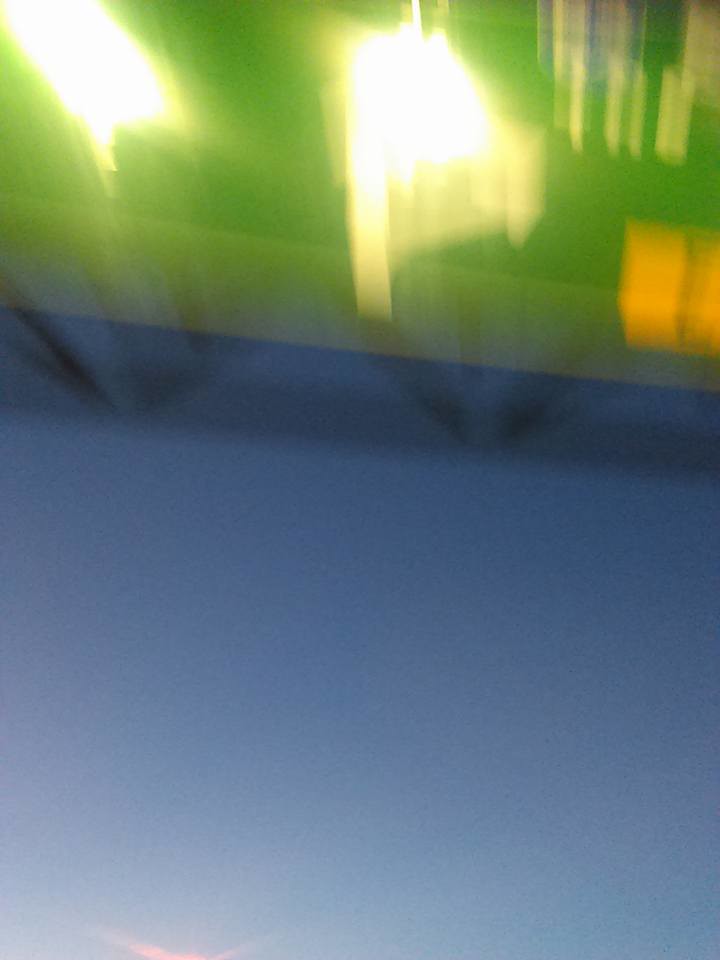In this very blurry yet vibrant photograph, the bottom portion is dominated by a smooth, swimming pool blue hue, suggesting either a surface or body of water. Above this, the composition transitions into a bright green area, suffused with intense, bright white lights emanating from the top, creating a significant amount of blur and visual obstruction. Towards the lower section of the green expanse, there is a conspicuous orange block that resembles a window, adding an element of structural intrigue. Directly above this, another rectangular shape appears, potentially another window, further contributing to the ambiguous, yet intriguing architectural narrative of the image.